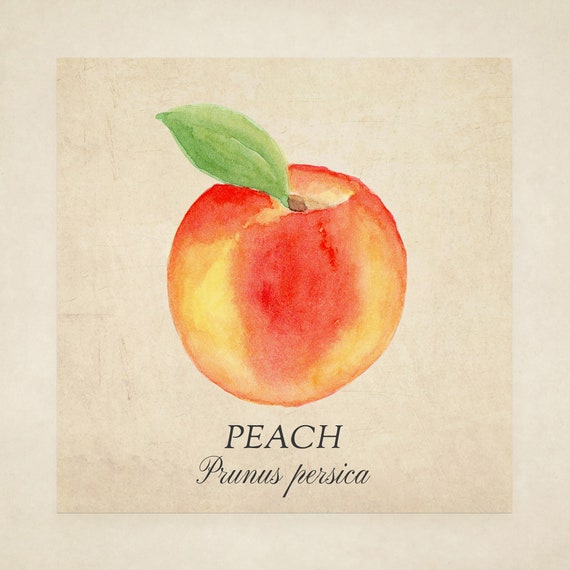The image depicts a detailed watercolor painting of a peach, situated on a deliberately distressed beige background with a lighter beige border. The peach features typical peach hues, blending yellows, pinks, and reds, and includes a single green leaf turned towards the left. Below the peach, in black text, "PEACH" is written in capital letters, with the scientific name "Prunus persica" elegantly rendered in cursive script underneath. The artwork is enclosed within a square frame set against a larger, light-tan square, enhancing its aesthetic presentation as a piece of art rather than a photograph.